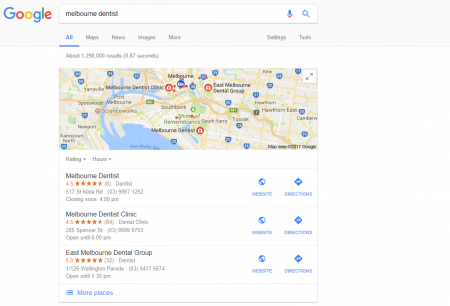The image showcases a Google Map focused on Melbourne, a city in Australia, highlighting several dentist locations marked with red pins. Each pin represents a different dental clinic in the area. Detailed information for each dentist is displayed below the map, including their ratings, number of reviews, addresses, hours of operation, contact numbers, and options for visiting their websites or getting directions. 

- One of the highlighted listings is "Melbourne Dentist," rated four and a half out of five stars based on eight reviews. 
- Another listing, "Melbourne Dentist Clinic," also has a four and a half out of five stars rating, but with 64 reviews. 
- "East Melbourne Dental Group" stands out with a perfect five out of five stars from 32 reviews.

The map itself includes visual elements such as bodies of water depicted in blue, major highways highlighted in yellow, and other significant roads marked with blue signs. Above the map, navigation options such as "Maps," "News," "Images," and "More," along with "Settings" and "Tools," are available, with "All" currently selected in blue. The entire setup provides a comprehensive overview of dental care options in Melbourne, making it easy for users to find and select a suitable dentist.